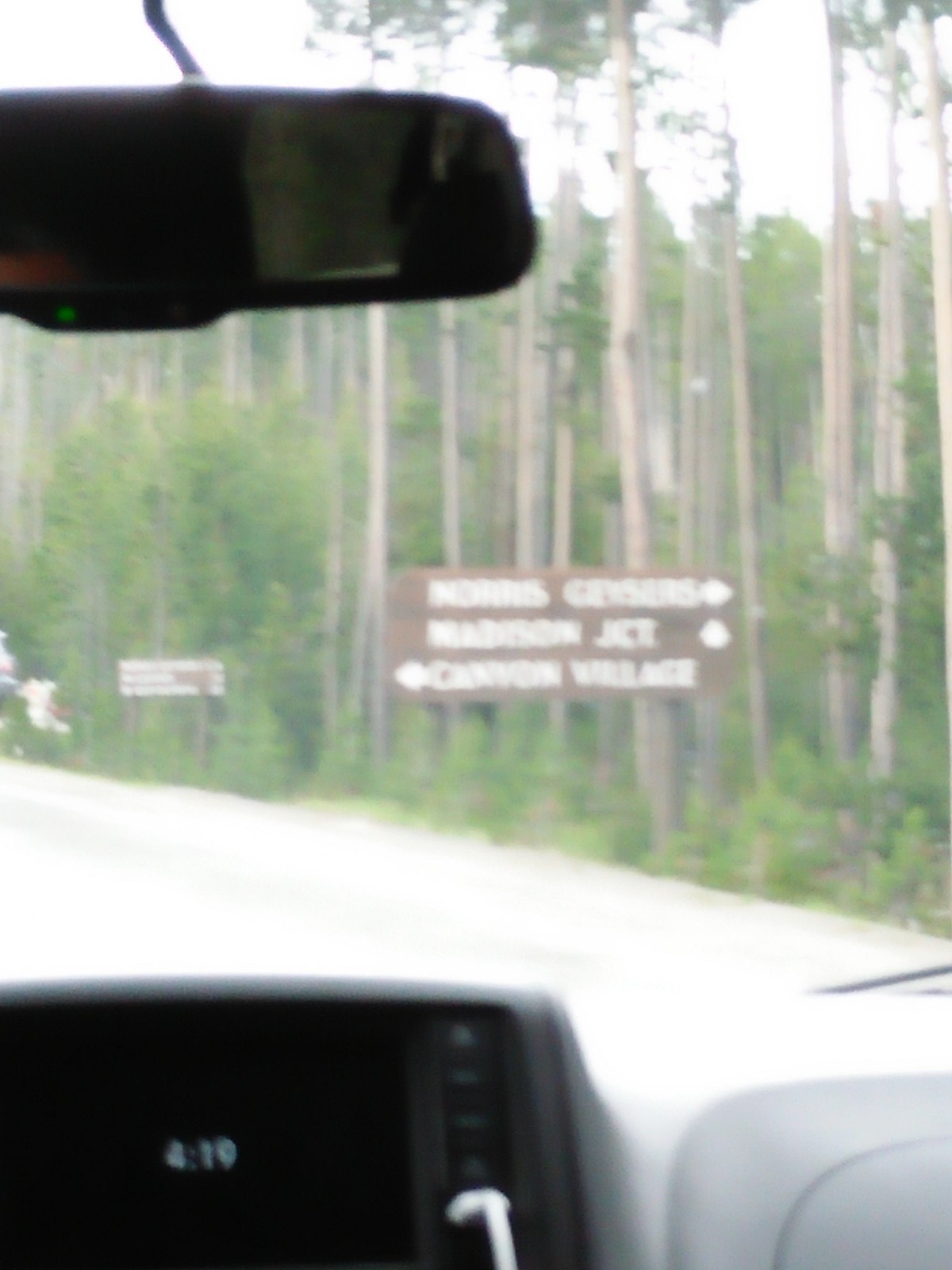This photograph, taken from inside a vehicle, appears to be shot from the back seat, capturing a point of view out through the front windshield. The car’s dashboard features a central control center with a clock displaying the time as 4:19. A USB port with a white charger plugged in is visible to the right of the dash. Above the dashboard, towards the left of the image, hangs a rear-view mirror. The interior of the car includes a visible portion of the glove compartment and is primarily gray in color.

Outside the windshield, the image provides a view of a wooded area filled with tall, slender tree trunks and dense green foliage. The road ahead appears washed out due to the lighting, giving it a white-gray appearance. Prominently, there is a brown wooden sign featuring white text and arrows pointing in different directions. Despite the blurriness, one can make out terms like "Norris Geysers" with an arrow pointing right, "Madison Junction" with an upward arrow, and "Canyon Village" with a right-facing arrow. Another smaller sign down the road also has text, but it is too blurry to discern the destinations indicated. The overall scene is slightly overexposed, giving the sky and parts of the road a washed-out appearance.